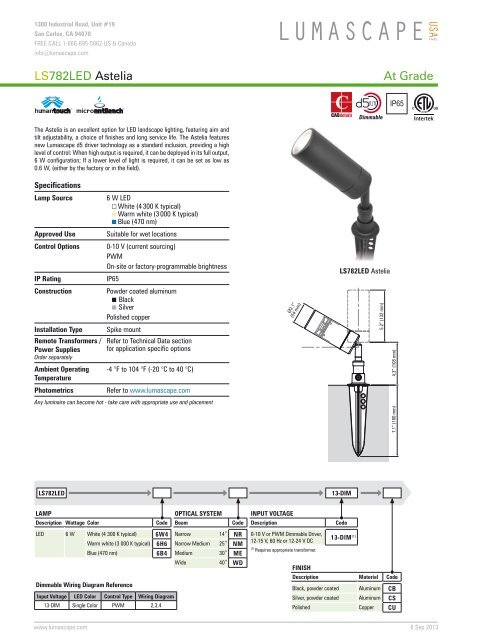This image is a screen capture of a web page detailing the specifications and features of the LS782 LED Astelia. The page is thoughtfully organized, with a chart on the left featuring a comprehensive list of specifications, including lamp source, approved use, control options, IP rating, construction, installation type, remote transformers, power supplies, ambient operating temperature, and photometrics. Each specification is concisely listed in black text on a white background, with occasional sections of text highlighted in light green for emphasis. The bottom segment of the page showcases flowchart schematics in black and white, providing visual aids for better understanding.

On the right side, the page is dominated by a vivid photograph of the LS782 LED Astelia. The product itself is depicted as a sleek, dark gray cylinder with an illuminating light emerging from the top. The cylinder is mounted at a diagonal angle on a matching black stem. Beneath the photograph, a detailed grayscale drawing illustrates the product's installation, showing how the bottom stem part is designed to extend into a solid surface, ensuring stability and proper placement. This well-structured layout provides a clear and detailed overview of the product.